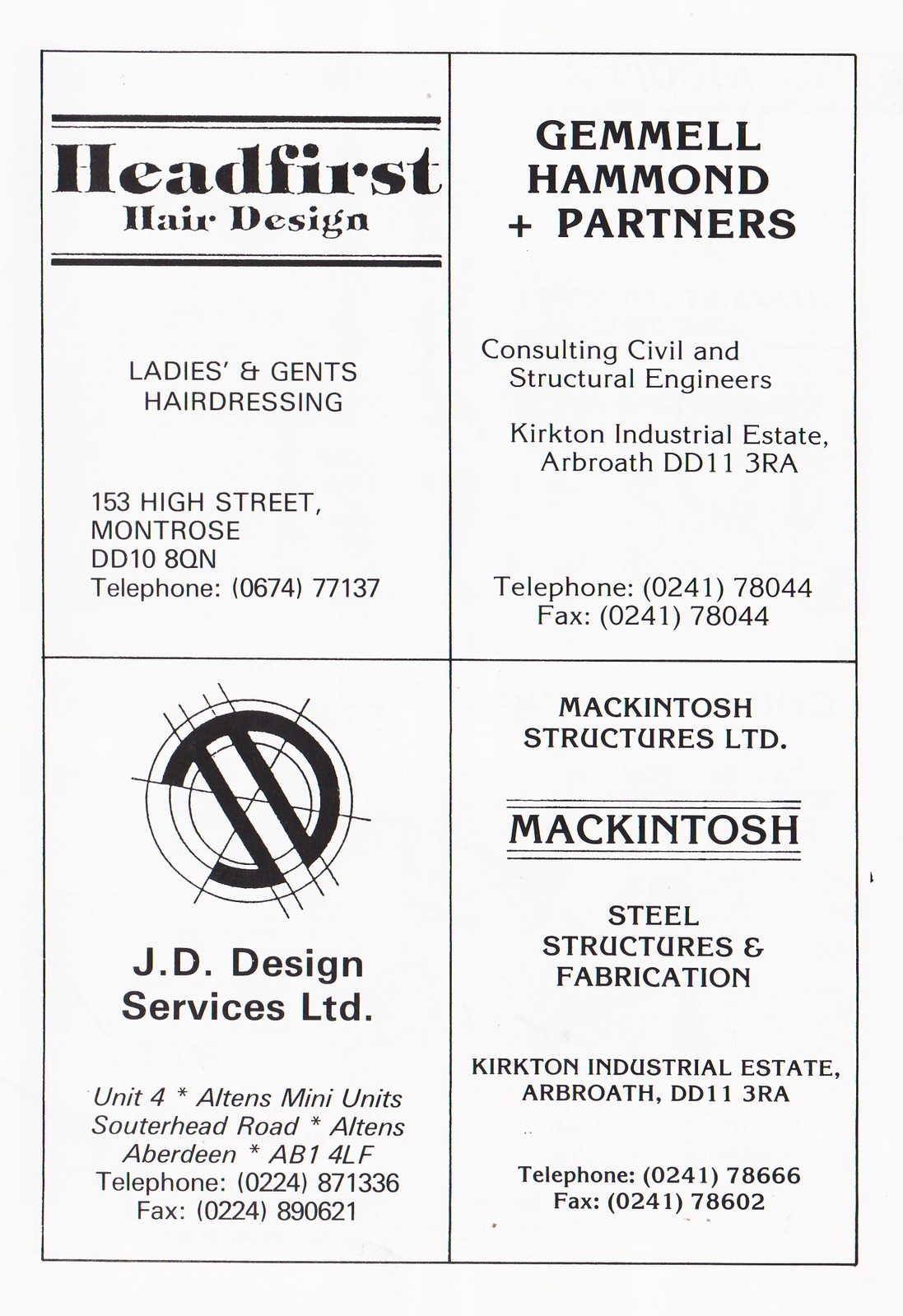The image showcases a four-section advertisement flyer with detailed information for various businesses. 

1. **Top Left Ad:** The ad promotes "Head First Hair Design," offering hairdressing services for both ladies and gents. It is located at 153 High Street, Montrose, DD10 8QN. For appointments and inquiries, the contact number is 067477137.

2. **Top Right Ad:** This ad is for "Gimel, Hammond and Partners," a consulting firm specializing in civil and structural engineering. Their office is situated at the Crickton Industrial Estate, DD11 3RA. They can be reached via telephone at 024178044, and the same number is used for fax.

3. **Bottom Left Ad:** Featuring a company logo, this ad represents "JD Design Services, LTD." Their office is located at Unit 4, Alton's Mini Units, Southerland Road, Alton's, Aberdeen, AB1 4LF. For contact, their telephone number is 0224871336, and the fax number is 0224890621.

4. **Bottom Right Ad:** This ad highlights "Macintosh Structures Limited," specializing in steel structures and fabrication. Their location is the Crickton Industrial Estate, DD11 3RA. They can be contacted via telephone at 024178666 and by fax at 024178602.